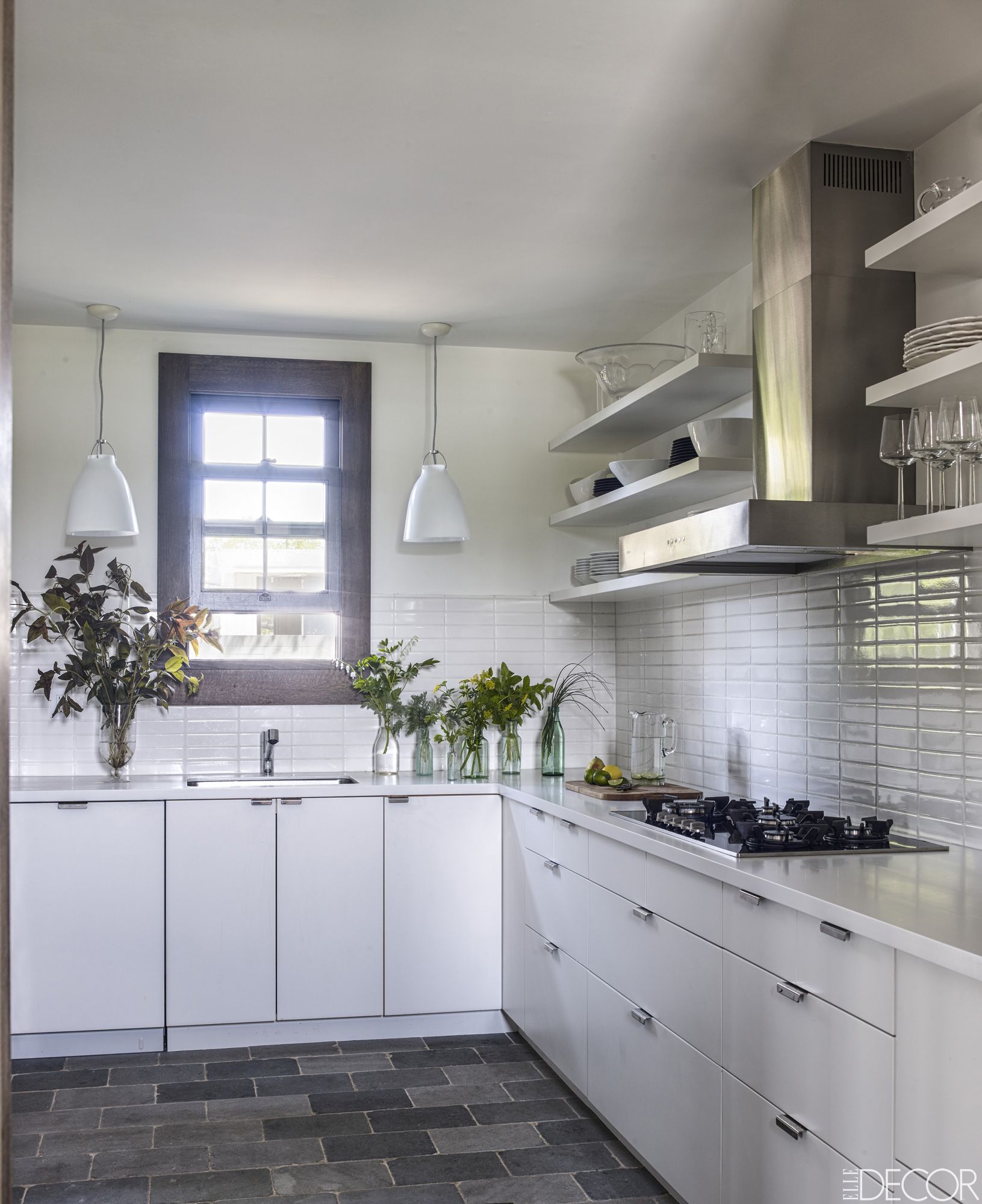This image captures a brightly lit, professionally photographed white kitchen interior. The kitchen features white walls and cabinetry, complemented by dark gray and light gray tiled flooring. To the left of the center is a window with brown borders, flanked by two minimalistic, conal-shaped lamps suspended from the ceiling. The cabinets below the window boast sleek metal fixtures akin to brushed aluminum, matching the modern sink faucet placed directly under the window.

The counter is adorned with a variety of plants in an array of clear glass vases, including one large leafy plant on the left and several smaller containers holding grassy-like plants, a pink flower, yellow flowers, and other greenery. A pitcher of water with lemons and limes rests on a cutting board near the side.

To the right of the sink is a black gas stove top with five burners, beneath a stainless steel exhaust hood. Surrounding this area, shelves are lined with a combination of kitchenware: a top shelf holding a crystal punch bowl, a middle shelf with three white bowls and some upside-down black bowls, and the bottom shelf furnished with plates and wine glasses. The room's layout is detailed further with cabinetry extending around the perimeter, featuring four drawers below the window and additional storage around the stove area, creating a cohesive and functional kitchen space.